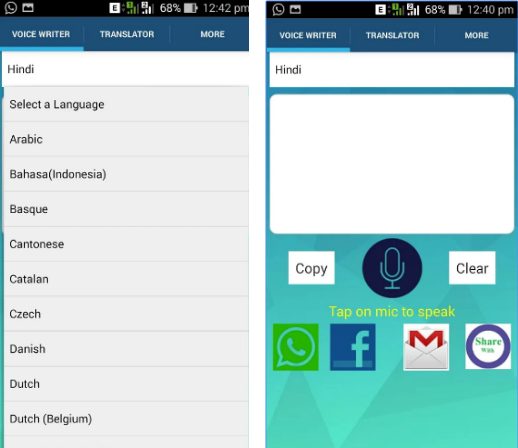The image displays a screenshot of a mobile device screen with several notifications and settings visible. At the top left, a WhatsApp notification is present alongside a gallery notification. A battery warning indicates the battery level is at 68%. The network status shows an EDGE connection, while the time in the top right corner is 12:42 PM. Below, the screen is divided into three sections labeled 'Voice', 'Writer', and 'Translator'. Various languages are listed, including Hindi (which is selected), Arabic, Bahasa (Indonesia), Cantonese, Catalan, Danish, and Dutch (Belgium). On the right side of the image, another screenshot highlights the Hindi language in the text input field.